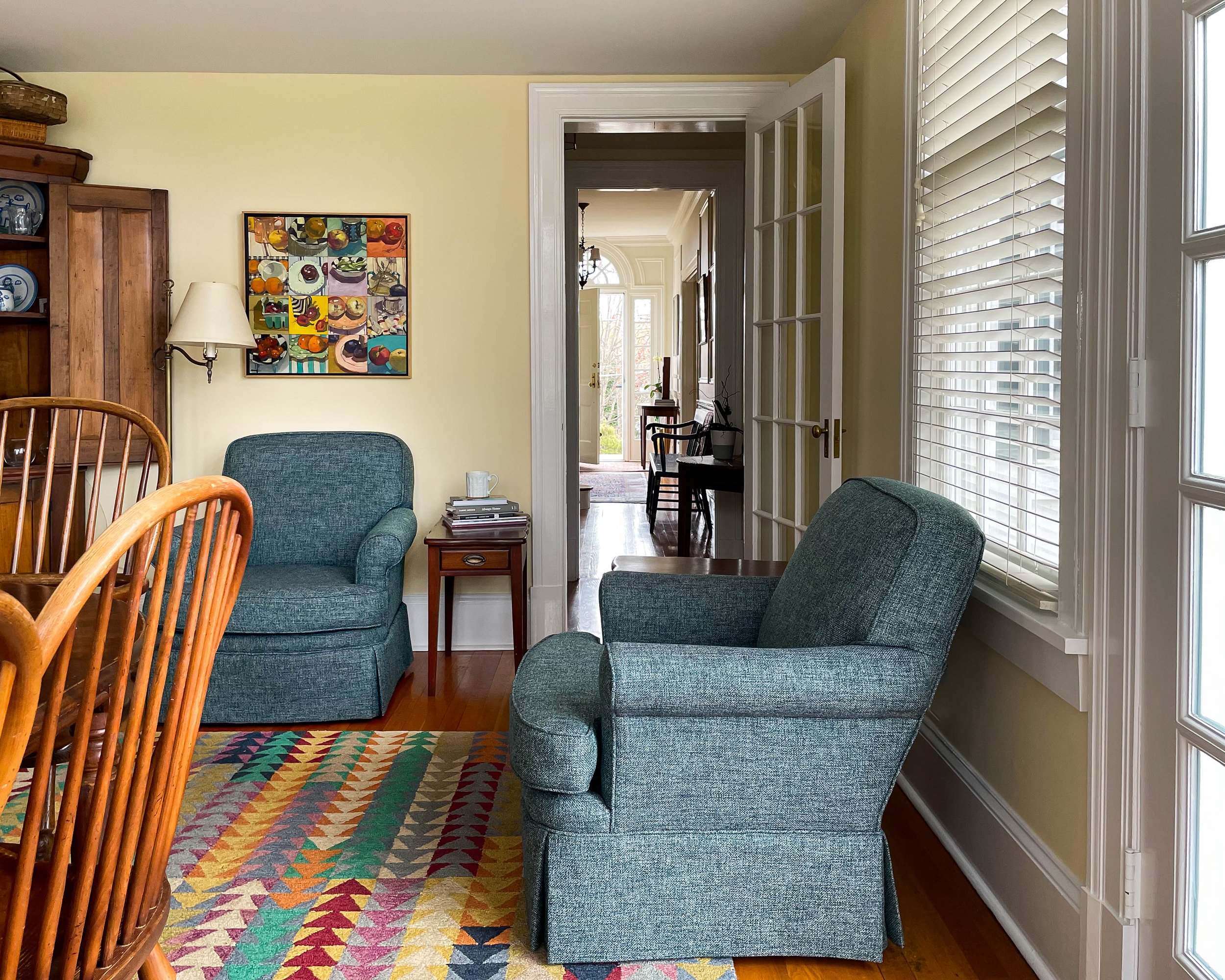The image depicts a cozy living room with light pastel yellow walls, featuring an open door in the background that presumably leads to the front door, where the edge of a chandelier is visible. Dominating the seating area are two armchairs; one centrally located in the foreground and another against the far wall, both providing a comfortable and inviting atmosphere. A medium-tone wooden floor is adorned with a beautiful pastel-colored rug characterized by a diamond and flying geese quilt pattern. In front of the seating arrangement sits a small coffee table, heaped with an assortment of books, adding to the room's lived-in charm.

To the left side of the image, a dining area with wooden chairs and a possible table can be glimpsed. An open wood cabinet is also visible, contributing to the room's rustic appeal. The far wall and the wall to the left feature artwork, with one painting appearing to be a food-themed montage. A window behind the armchair on the right bathes the room in natural light, further emphasized by a tall window visible through an open door on the right, which leads to another room or hallway. Adding a touch of elegance, a lamp hangs on the wall across from the viewer. The overall aesthetic of the room is warm and inviting, combining practicality with artistic touches.